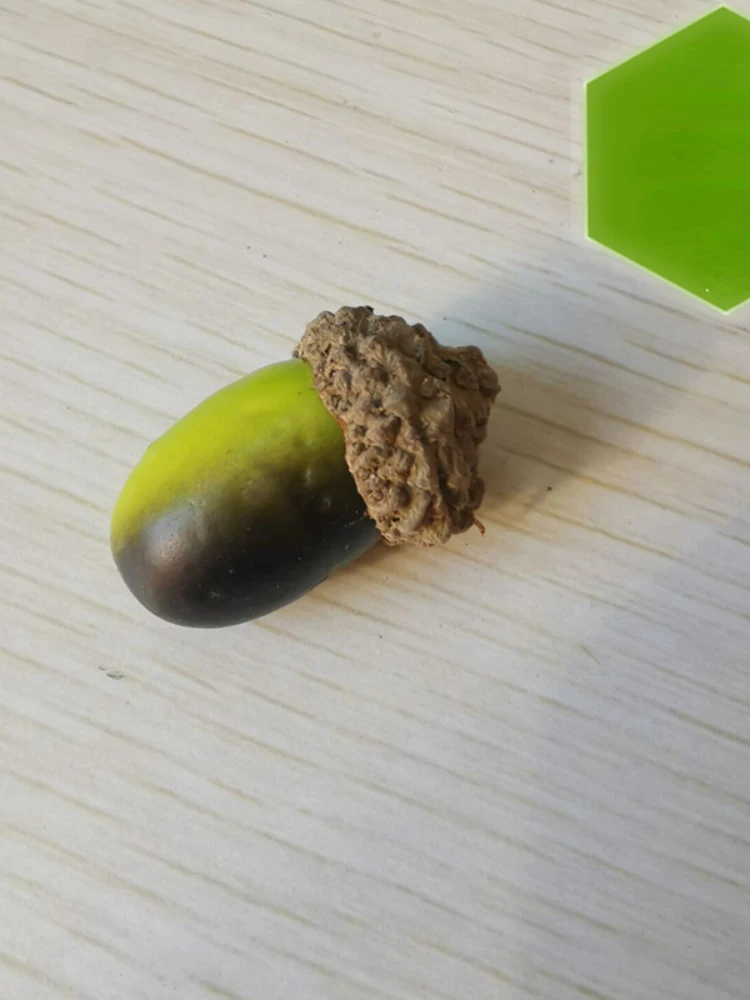The image features a decorative acorn positioned on a pine-colored wooden table with a sandy gray hue accented by darker stripes. The acorn, centrally placed and not occupying much space, features a light green top and a darker green nut body, with a brown, textured cap that has indents to mimic a real acorn, tapering into a rounded, knob-like point. In the top right corner of the photograph, there is a green cube or block, though its exact nature is unclear. The acorn casts a faint shadow behind it, and the green cap points toward the upper right, creating a subtle diagonal line from the top right to the bottom left of the composition. The close-up perspective emphasizes the acorn’s minute details against the understated wooden backdrop.